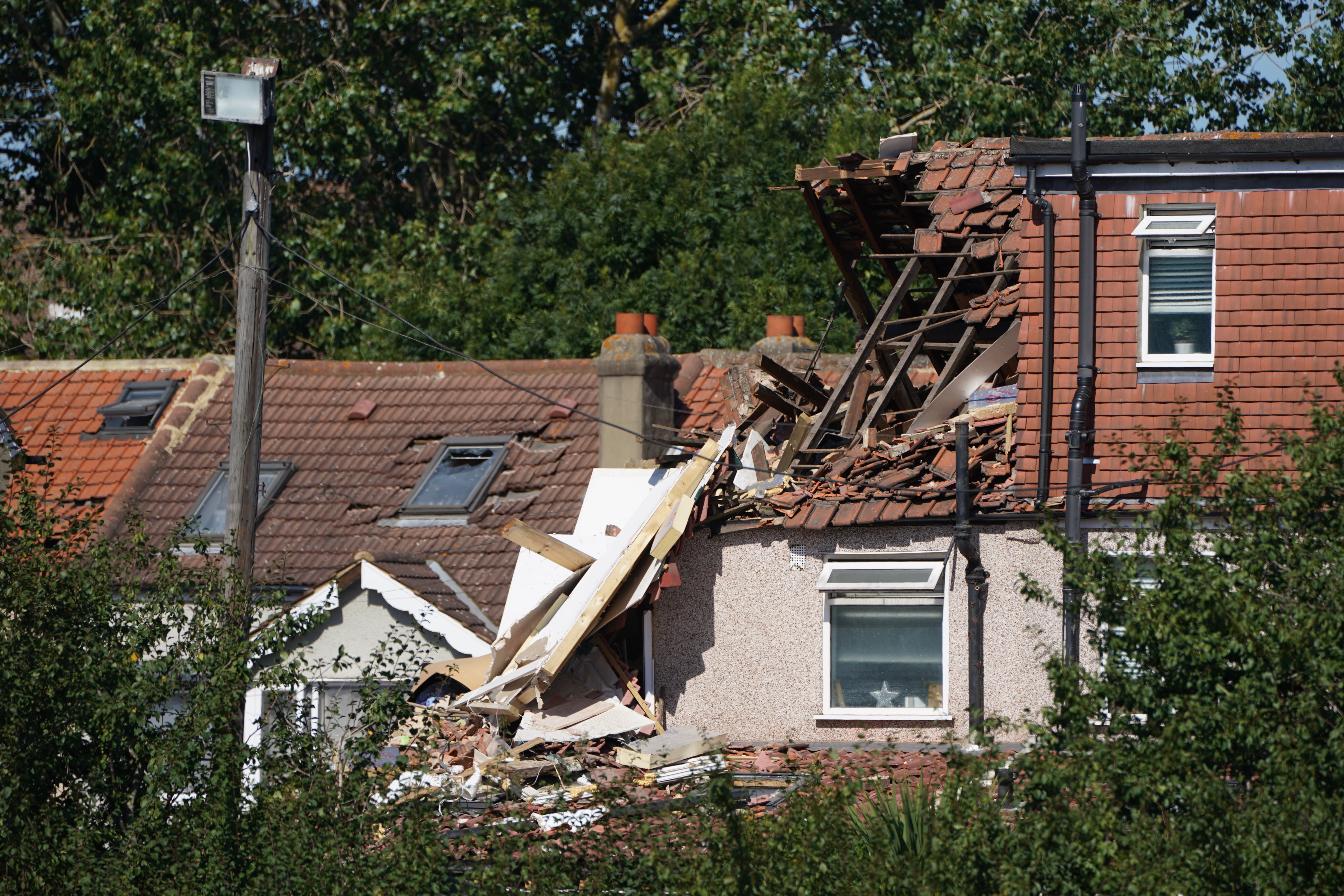The image depicts a scene of structural damage, primarily focusing on a severely damaged two-story house. In the foreground, there's a row of shrubs or small trees, and just behind that, an electrical pole is partially visible. The most prominent structure is a house where the left wall is destroyed, exposing significant debris on the second floor. The left portion of the roof is missing, revealing the frame of the house and scattered shingles. Surrounding this house are additional buildings that also exhibit damage, albeit less severe. These structures have broken windows, including a skylight-type window, and missing or misplaced shingles. Beyond these buildings, tall trees obscure much of the sky. There are additional background elements, such as more trees, big poles with lights on top, windows, and various plants. The overall scene is one of significant destruction, highlighted by the completely demolished roof and extensive debris scattered throughout the area.